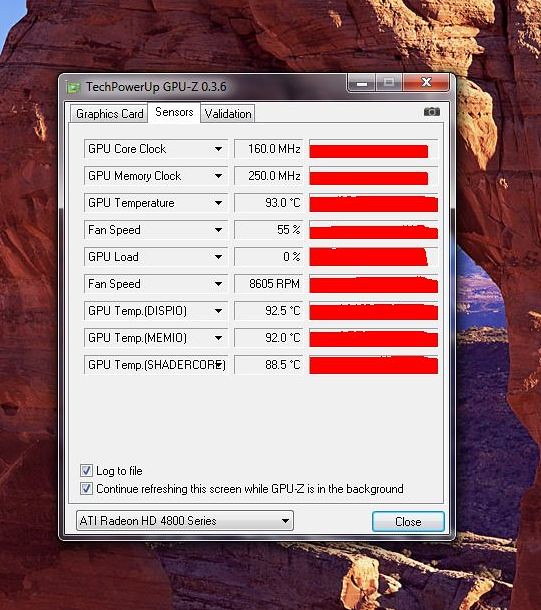The image displays a computer screen with an Arizona-style desert rock formation as the background. In the foreground, there is an open software window titled "TechPowerUp GPU-Z 0.3.6," focusing on the specifications and performance metrics of a graphics card. The window has three tabs: Graphics Card, Sensors, and Validation. The Sensors tab is currently selected, detailing various metrics such as GPU Core Clock, GPU Memory Clock, GPU Temperature (93°C), Fan Speed (55%), GPU Load (0%), and Fan Speed (8605 RPM). Additional readings show different GPU temperatures, including 92.5°C, 92.0°C, and shader core temperature at 88.5°C. The graphics card is identified as an ATI Radeon HD 4800 series, selectable via a drop-down menu. At the lower right corner of the window, a button labeled "Close" is available to exit the screen. Adjacent to these readings, a red bar graph visually represents some of these metrics, and options to log data and refresh the screen are also present.